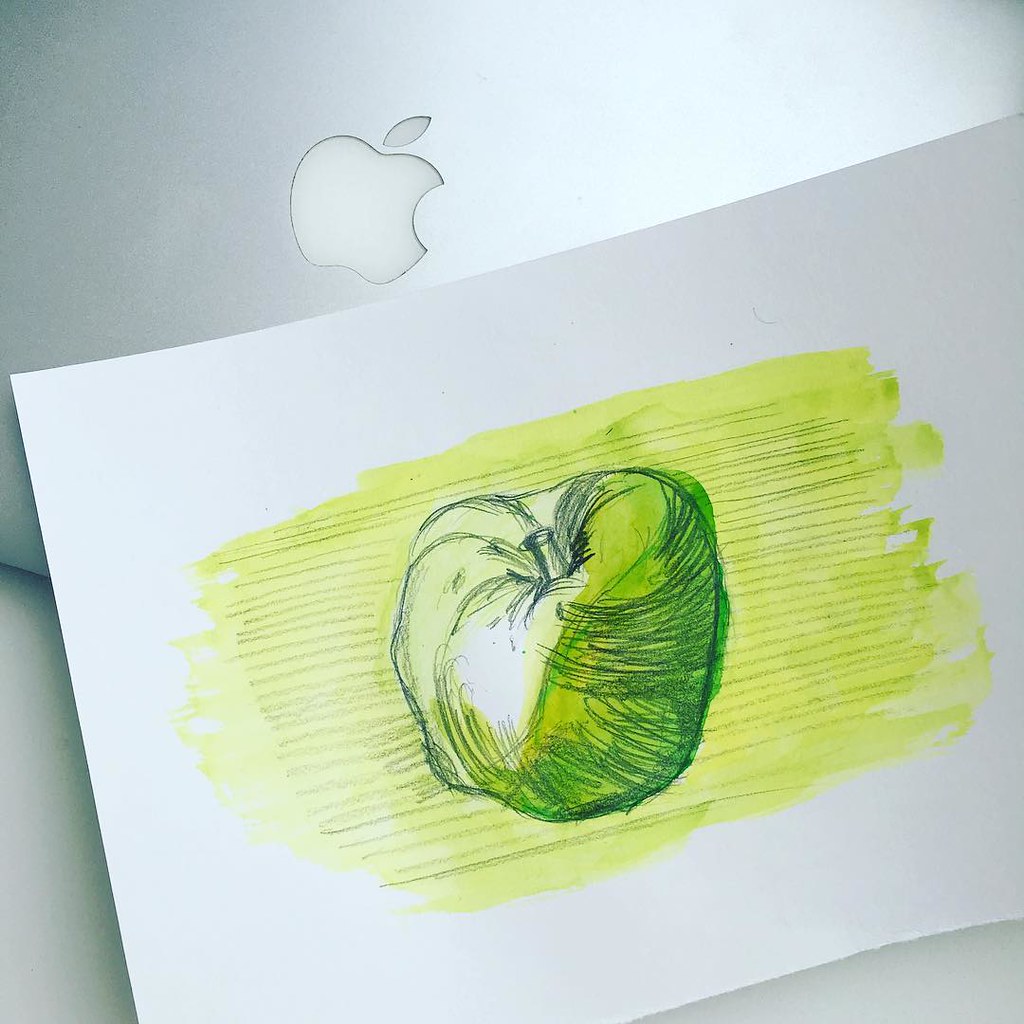The image features a piece of paper containing a hand-drawn sketch of an apple rendered in either blue or black ink. The apple appears aged and shriveled, with intricate details giving it a realistic, albeit weary, texture. Hovering above the sketch is a closed silver Apple laptop, its iconic illuminated apple logo clearly visible, providing a stark contrast to the depicted fruit.

The apple in the sketch is predominantly colored with streaks of a yellowish-green highlighter, creating an uneven, somewhat distressed appearance. The light source is suggested by a small, uncolored shiny spot on the apple, representing a gleam of reflected light. The application of the highlighter has caused the ink to smear slightly, adding to the worn and angry demeanor of the apple.

Overall, the combination of the old, shriveled apple sketch and the sleek, modern laptop aims to draw a visual and thematic contrast between age and modernity, nature and technology. The sketch evokes a subtle, almost unsettling emotion, giving the impression of an 'angry' apple.